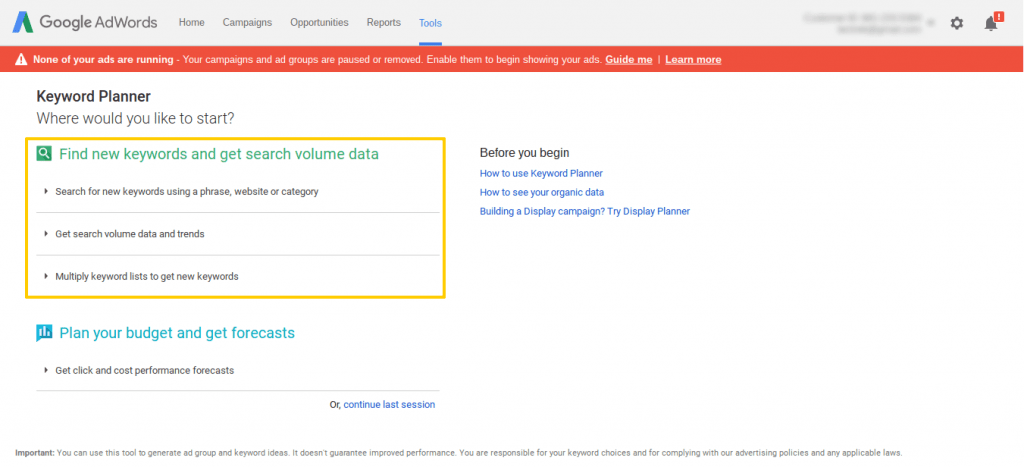The image is a screenshot of the Google AdWords website. The layout is approximately two and a half to three times wider than it is tall. At the top, there is a light gray bar stretching from left to right. In the upper left corner, an upside-down V-shaped logo is present, with its left half colored medium blue and the right half dark green, representing the Google AdWords logo. Next to the logo, the text "Google AdWords" is displayed, followed by navigation menu options including Home, Campaigns, Opportunities, Reports, and Tools. The "Tools" option is written in blue and underlined, indicating the current section.

In the upper right section, there's a blurred-out login area, accompanied by a settings icon and a bell notification icon with the number one. Below the top bar, a warning message is displayed in white text on a red background. Directly beneath this, the header "Keyword Planner" is shown in bold on a white background. Underneath this header, the text in a regular font asks, "Where would you like to start?"

The main section below is highlighted with a yellow rectangle, drawing attention to a dark green box containing a white magnifying glass icon. To the right of this icon, the text reads: "Find new keywords and get search volume data," indicating the available options within this section.